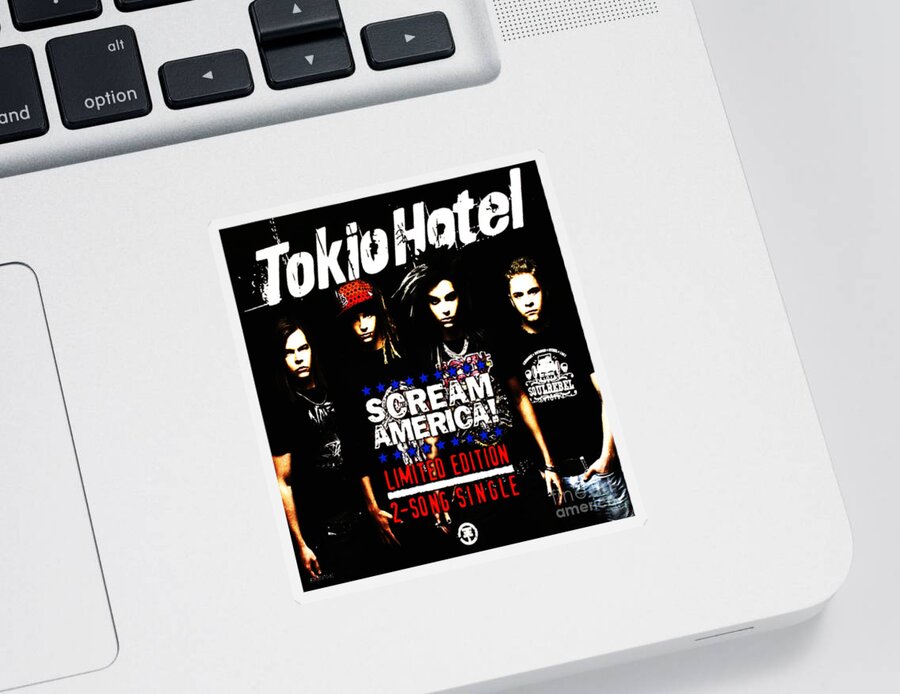This image captures the bottom right corner of a laptop, revealing a portion of the mouse pad on the left and the visible keys on the keyboard, including the 'AND' key, the 'ALT' key (also labeled as the 'option' key), and the arrow keys. At the top right corner of this section, a speaker is evident. The laptop prominently displays a sticker of the band Tokyo Hotel. The sticker features the four band members, who are all dressed in black. The member second from the left stands out with a red hat, while the one next to him has notably long hair. All band members appear pale and are not smiling, with the member on the left displaying a particularly stern expression. The poster includes the title "Tokyo Hotel," with "Scream America!" written in bold white letters, accented by blue stars above and below the text, and a red inscription below stating "Limited Edition Two-Song Single."